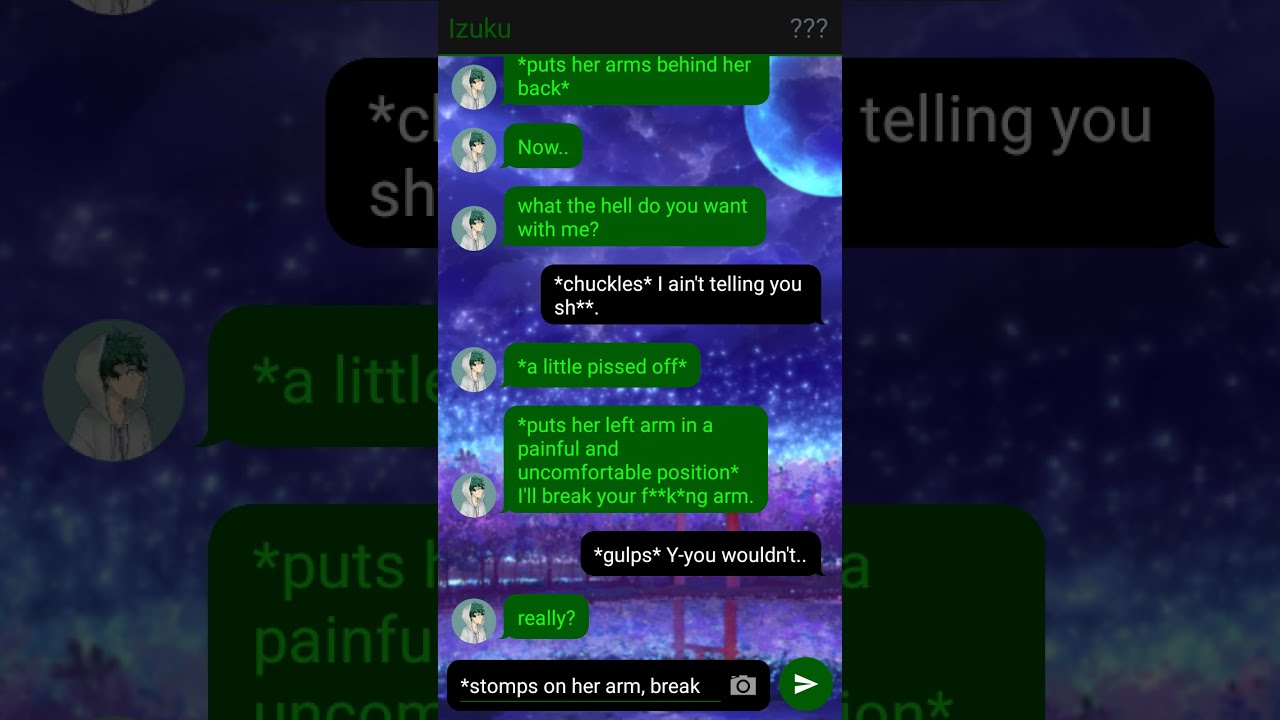The image is a detailed screenshot of a text conversation on what appears to be an Android device, indicated by the green text bubbles. On the left, small circles display an avatar resembling a boy with dark hair and a hoodie, though the details are indistinct. The conversation reads as follows: 

1. In green: *puts her arms behind her back* 
2. Green: "Now, what the hell do you want with me?" 
3. In black, replying: *chuckles* "I ain't telling you anything."
4. Green: *a little pissed off* "I'll break your f***ing arm."
5. Black: *gulps* "You wouldn't."
6. Green: "Really?"
7. Black: *stomps on her arm* "Break."

The dialogue portrays a tense confrontation, with the avatar on the left threatening and ultimately enacting physical harm on the other person in the chat. The black and green text colors help differentiate between the two participants in this heated exchange.